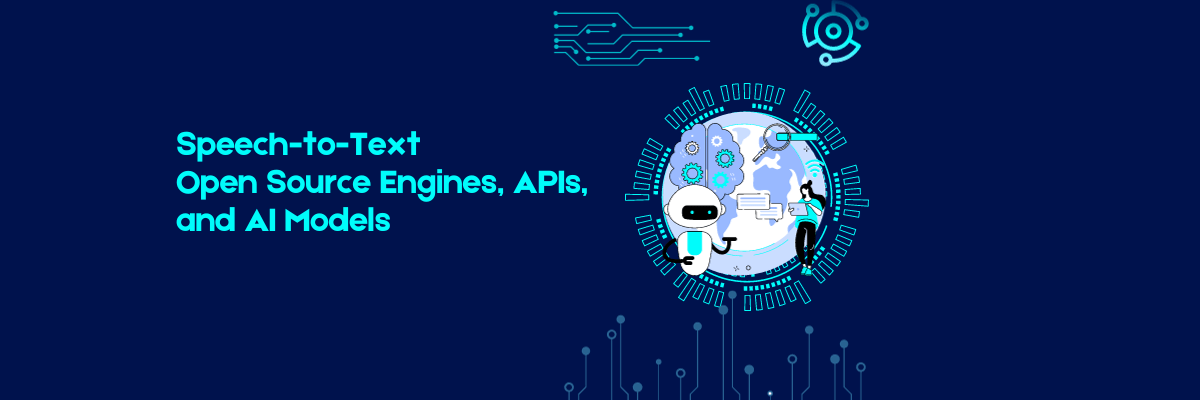This image resembles an advertisement, divided into two main sections. The left side features a dark purplish-blue background with teal-green lettering that reads, "speech to text, open source engines, APIs, and AI models." The right side contains a circular design showcasing various visual elements, including a white chatbot with a black face and arms, a globe highlighting the African continent, a brain intertwined with gears, a magnifying glass, and a girl writing in a notebook. The overall color scheme of the visuals is primarily white and light blue. This advertisement evidently promotes AI and speech-to-text technologies, highlighting the components and tools associated with these innovations.